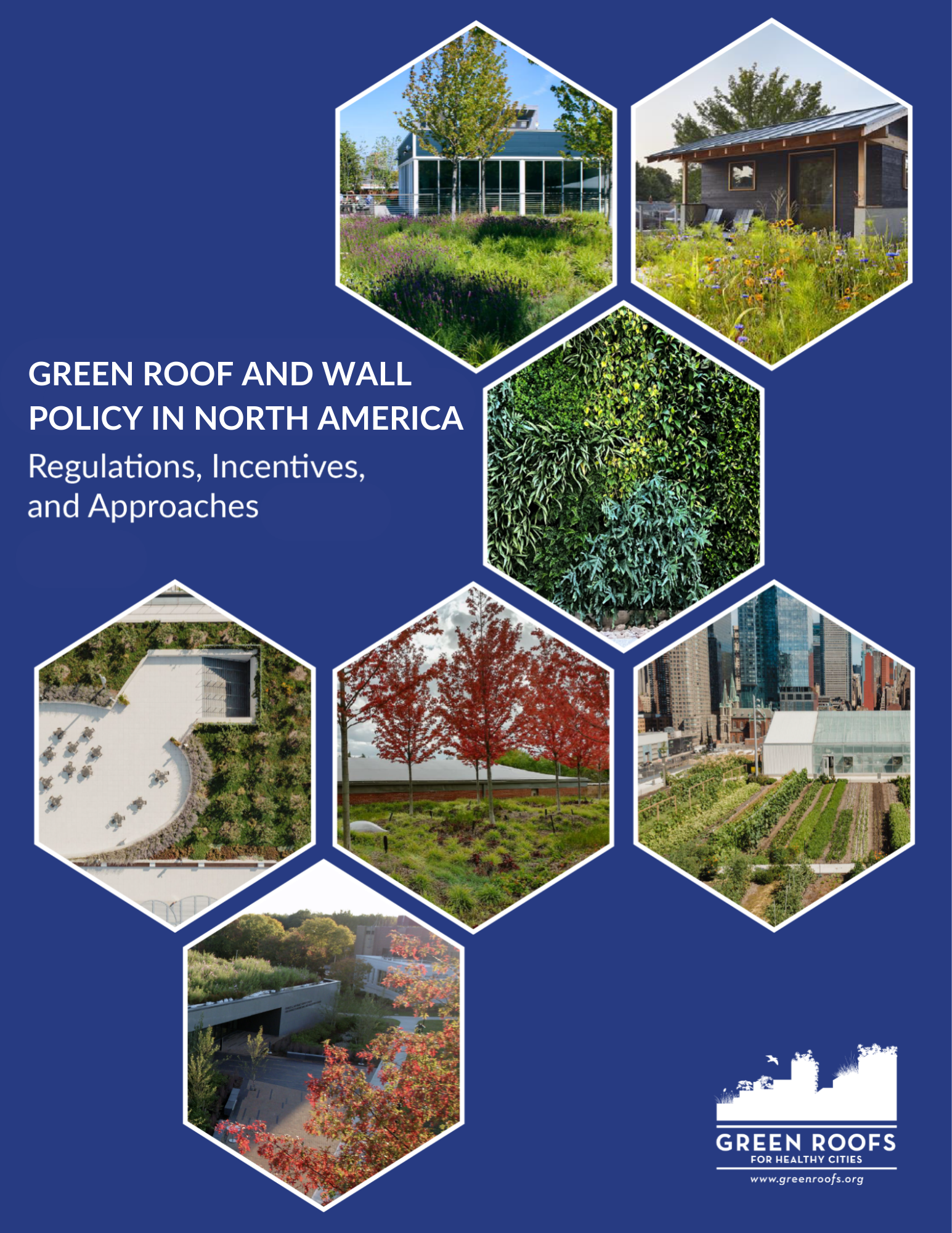This advertisement flyer for "Green Roof and Wall Policy in North America: Regulations, Incentives, and Approaches" by Green Roofs for Healthy Cities (greenroofs.org) is set against a blue background. The flyer features a geometric grid of hexagon-shaped photographs that display various outdoor images, mostly depicting rooftops and vibrant greenery, including plants, shrubs, and landscaped areas. The hexagons are meticulously arranged to border each other, creating a cohesive visual effect. The white, all-caps text includes both the main headline and additional information about the policy and approaches to integrating green roofs and walls, emphasizing sustainable urban landscaping. The overall design is eye-catching and expertly crafted to convey the initiative's goals and benefits visually.